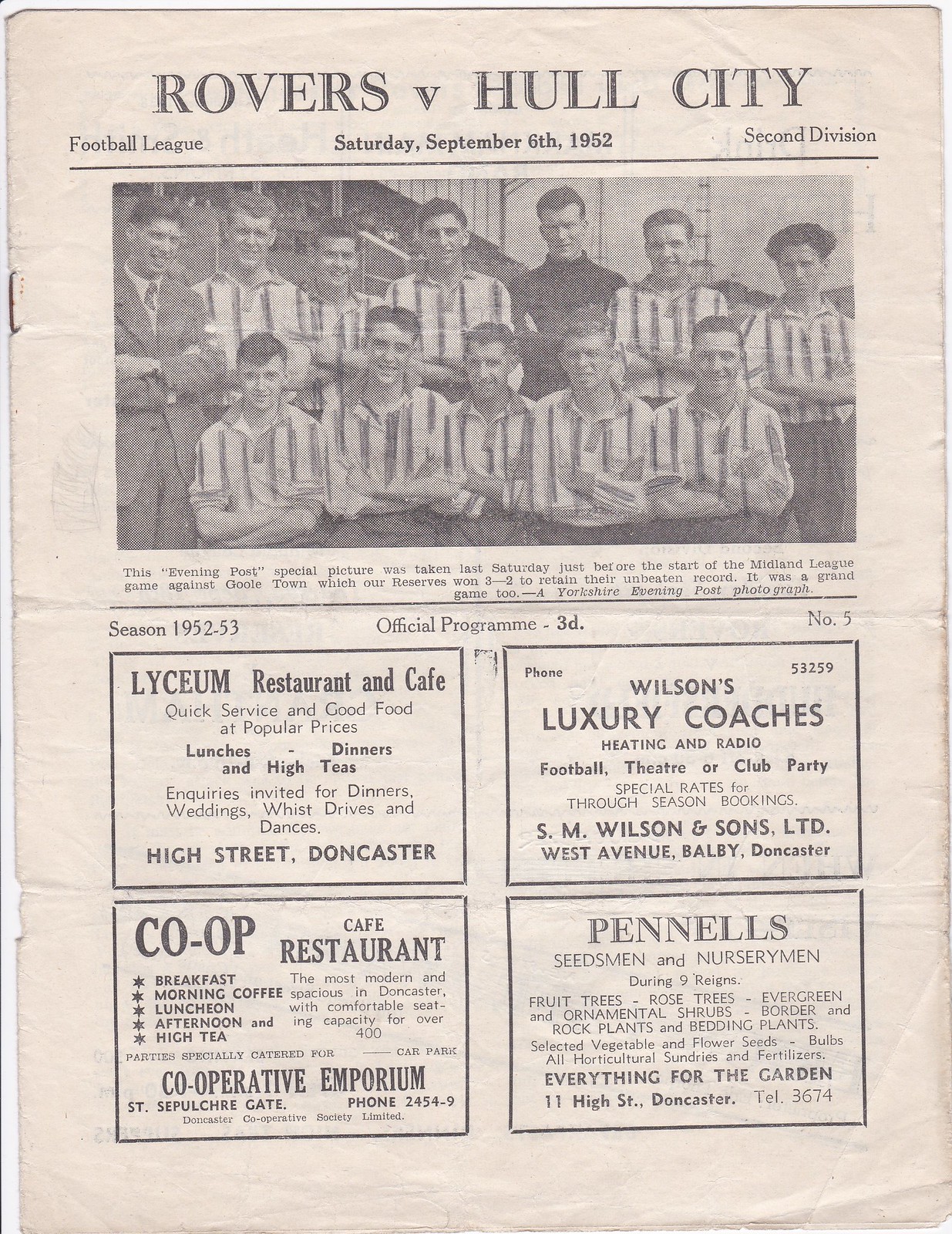The image appears to be a scanned page from an antique newspaper, dated Saturday, September 6, 1952. At the top, it reads, "Rovers v. Hull City Football League, 2nd Division." Below that, there is a black and white photograph featuring two rows of men in uniforms, arms crossed and smiling, captured just before the start of the Midland League game against Gould Town, which the reserves won 3-2 to retain their unbeaten record. The caption under the photo declares it a "Yorkshire Evening Post special picture," taken last Saturday. The text also notes that the image is part of the "Season 1952-53 Official Program, 3D, No. 5."

The lower portion of the page consists of four distinct advertisements:
1. **Lyceum Restaurant and Cafe**: Quick service and good food at popular prices. They offer lunches, dinners, and high teas, and cater events like weddings and dances. Located on High Street, Doncaster. 
2. **Wilson's Luxury Coaches**: Providing heating and radio services for football, theater, or club parties, with special rates for season bookings. Contactable via phone at 53259, located on West Avenue, Balby, Doncaster.
3. **Co-op Cafe Restaurant**: Serving breakfast, morning coffee, luncheon, afternoon, and high tea, in a modern and spacious establishment with seating for over 400. Located at Cooperative Emporium, St. Sepulchre Gate, Doncaster.
4. **Pinnell's Seedsmen and Nurserymen**: Offering a variety of garden supplies including fruit trees, rose trees, evergreen and ornamental shrubs, select vegetables, flower seeds, bulbs, and fertilizers. Located at 11 High Street, Doncaster, contactable via phone at 3674.